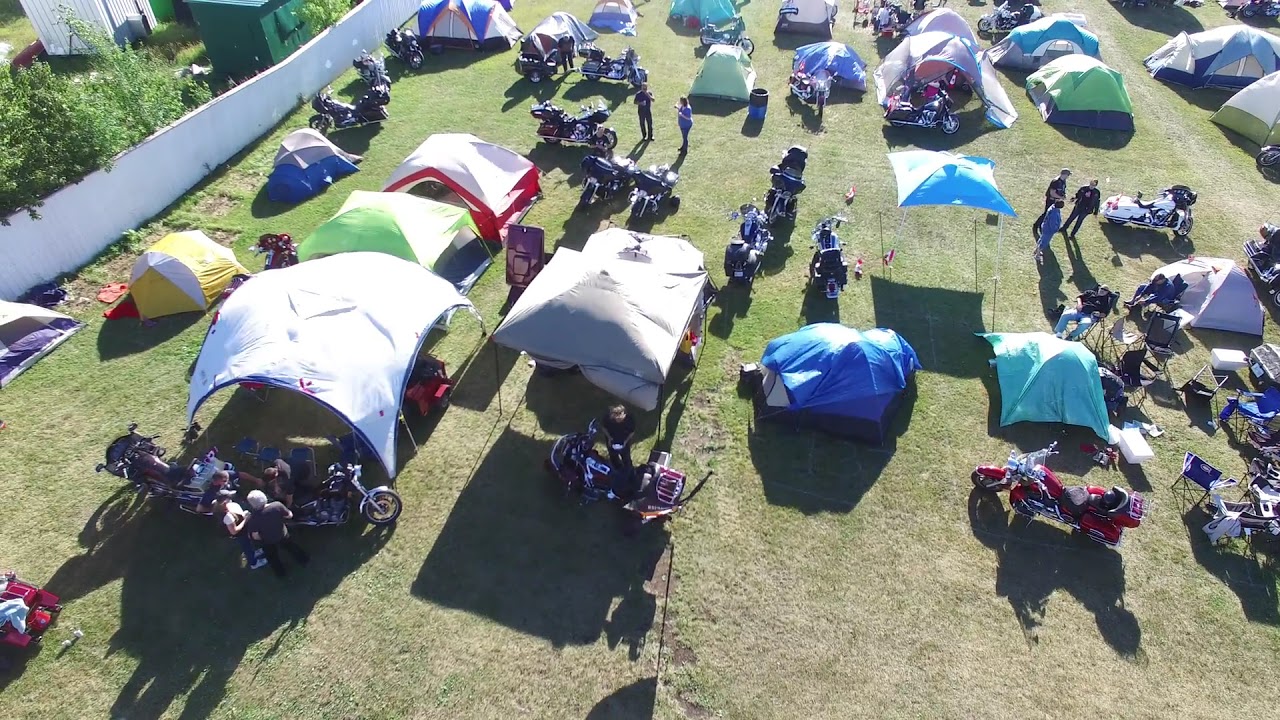This aerial photograph, taken from approximately 100-200 feet above, reveals a lively campsite likely hosting a motorcycle gathering. The scene showcases a large, open grassy area dotted with around 20 tents and canopies, ranging in colors such as blue, green, white, red, and gray. Motorcycles, in shades of red, chrome, black, and blue, are parked beside each tent, indicating the campers are motorcyclists, possibly preparing for a night’s rest. People can be seen milling about, conversing in small groups, and inspecting the motorcycles. A white fence runs along the left side of the image, behind which lies an overgrown garden and possibly a shed. The canopies, some without walls, are supported by thin poles, casting distinct shadows on the grass, suggesting it is late in the day. Small trees pepper the left side of the image, and the light blue canopy in the center-right casts a notable square shadow. Overall, the bustling yet cozy atmosphere suggests a social event filled with camaraderie among motorcycle enthusiasts.